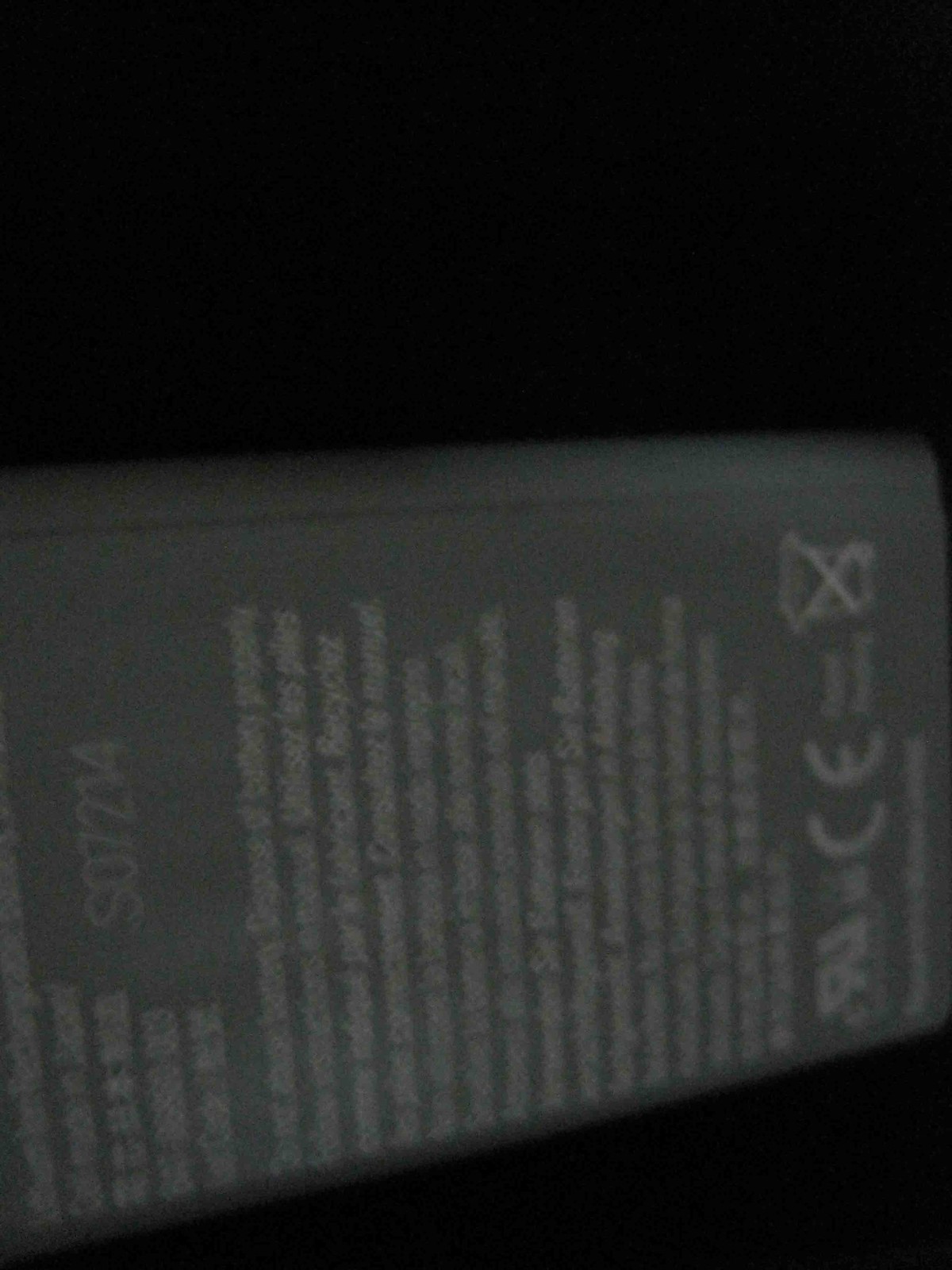This is a photograph of an instruction manual, visibly taken under poor lighting conditions, resulting in a very dark and out-of-focus image. The manual, presumably for an appliance or electronic device, is almost indiscernible due to the glare affecting the readability of the printed text. The only legible part is a partial identification number that appears to be "S-O-714," although some characters are unclear. The background is entirely black, emphasizing the limited visibility of the document and the surrounding area.